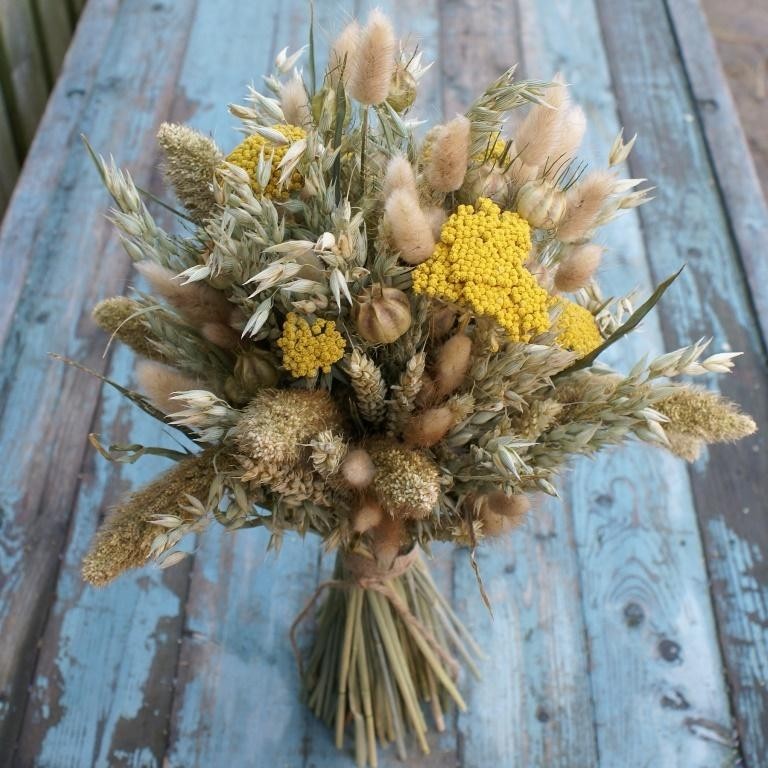The photograph captures a dried flower bouquet arranged on a weathered, distressed wooden table. The bouquet stands upright without the aid of a vase, bound together at the stems by string. The tableau is rustic, evoking a country charm with flowers that seem gathered from a farm or field. The dried flowers are primarily in shades of tans, browns, and beiges, interspersed with yellow baby's breath that adds a pop of color. Some green leaves and wispy cat's tail plants peek out from the arrangement, and a distinctive tan bulb-like wildflower contributes to its unique appearance. The wooden table beneath has a chipped, silvery gray paint that adds to the rustic aesthetic, with patches of unpainted wood visible. The overall effect is a beautiful, natural, and earthy composition.